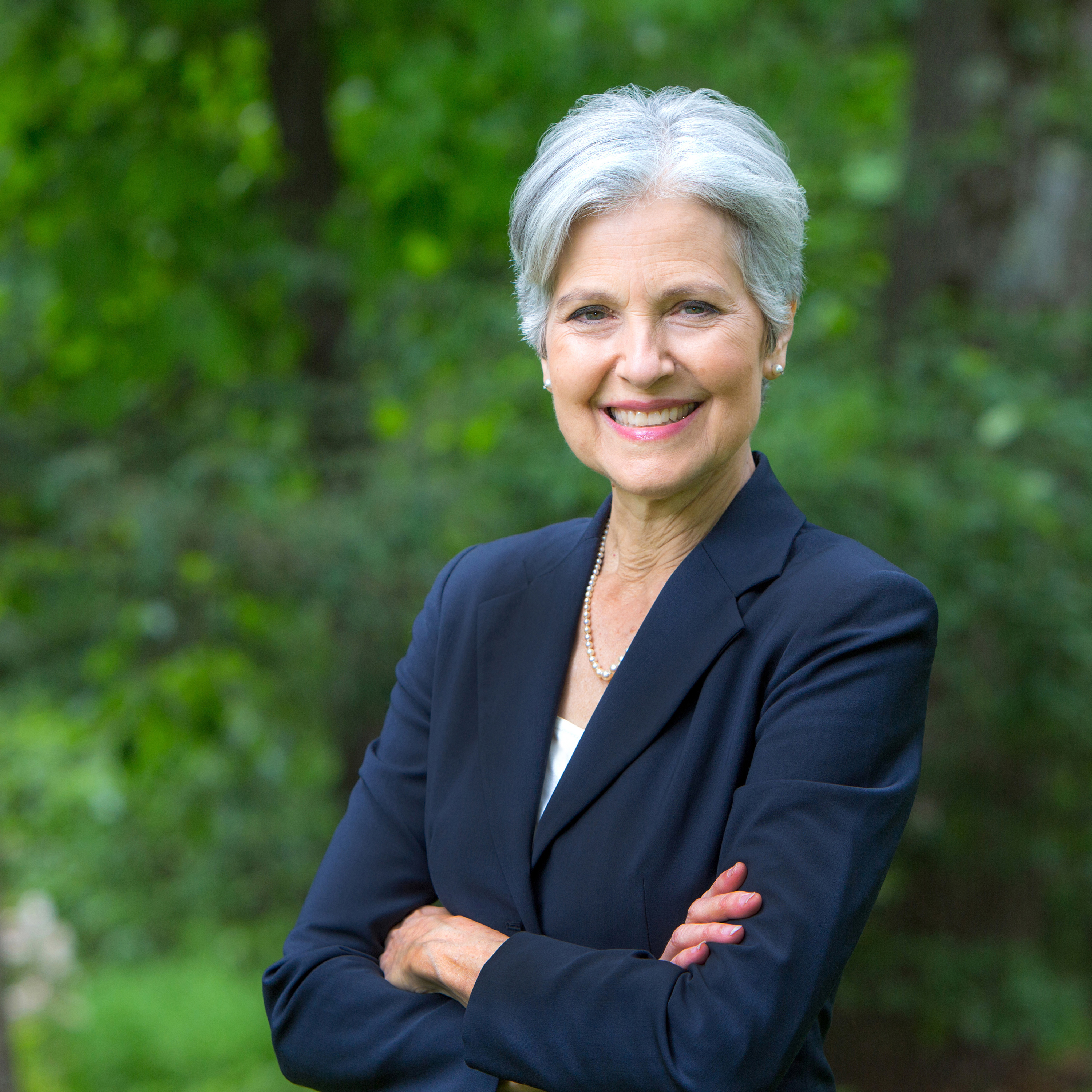This detailed portrait captures an elderly woman, likely in her 60s or 70s, standing outside against a backdrop of blurry, green foliage, suggestive of trees. She is photographed from the waist up, directly facing the camera with a wide, cheerful smile. Her white hair is parted in the middle and styled to a medium length, giving her a warm and approachable demeanor. She is impeccably dressed in a dark blue blazer over a white blouse, accentuated by a classic pearl necklace and matching pearl earrings. The woman's arms are confidently crossed in front of her, exuding a sense of calm and contentment. Her makeup is subtle yet elegant, featuring pink lipstick that complements her overall appearance. This image, dominated by shades of green and blue, beautifully captures the joyful essence of the subject amidst a serene, natural setting.